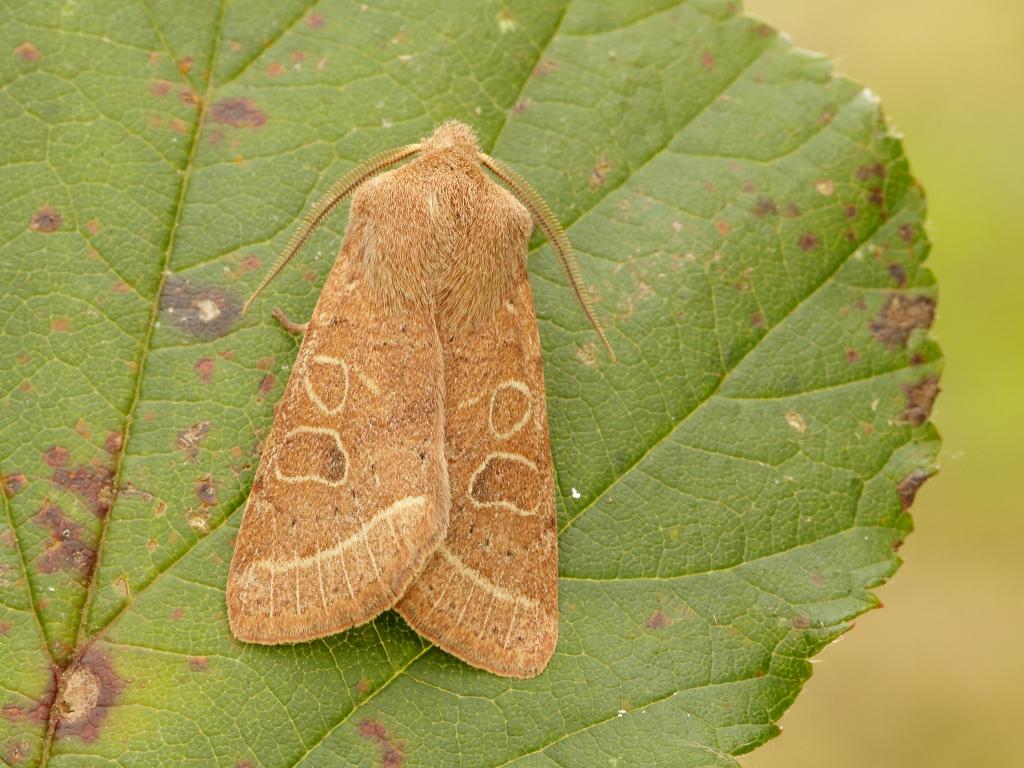A close-up photograph showcases a captivating scene where the background is an artfully blurred blend of tan hues with a touch of green, possibly from an out-of-focus leaf. Dominating the composition is a large, medium green leaf with scattered brown patches along its right edge and central vein. The true focal point, however, is a strikingly beautiful tan moth perched prominently on the leaf. The moth's light tan wings, adorned with irregularly shaped ovals, exude an understated elegance. The wing tips display intricate, lighter-colored lines that add to its delicate appearance. Long, ribbed antennae stretch gracefully from the moth’s head, completing its ethereal look. One can only imagine the splendor of this moth with its wings fully spread.